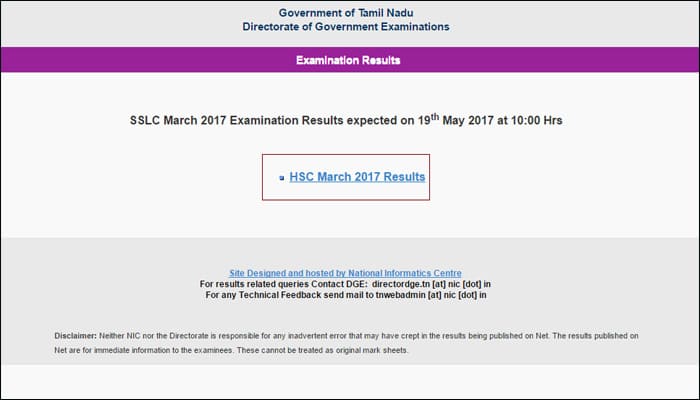The image depicts an official document presenting the test results notification for a student who undertook government examinations in Tamil Nadu, India. The document layout is in a landscape orientation with a thin black border enclosing the content.

At the top, there's a light gray rectangular banner displaying the text: "Government of Tamil Nadu, Directorate of Government Examinations." Below this, housed within a purple rectangular banner with white font, it reads: "Examination Results."

Following these headers is a larger rectangular section providing specific information about the results release. It announces: "SSLC March 2017 examination results expected on 19th May 2017 at 10:00 HRS."

Beneath this announcement is a magenta button containing a blue hyperlink text: "HSC March 2017 results," indicating a clickable link for accessing those results.

Towards the bottom of the image, another gray rectangular section includes additional information and a hyperlink pertaining to the website designed and hosted by the National Informatics Center. This section ends with details for results-related queries.

In essence, this document serves as a notification for the student to access their SSLC March 2017 examination results, which were expected to be available on May 19, 2017, at 10:00 AM. The document emphasizes its formal nature by specifying the state-run governing body and technical support provided.